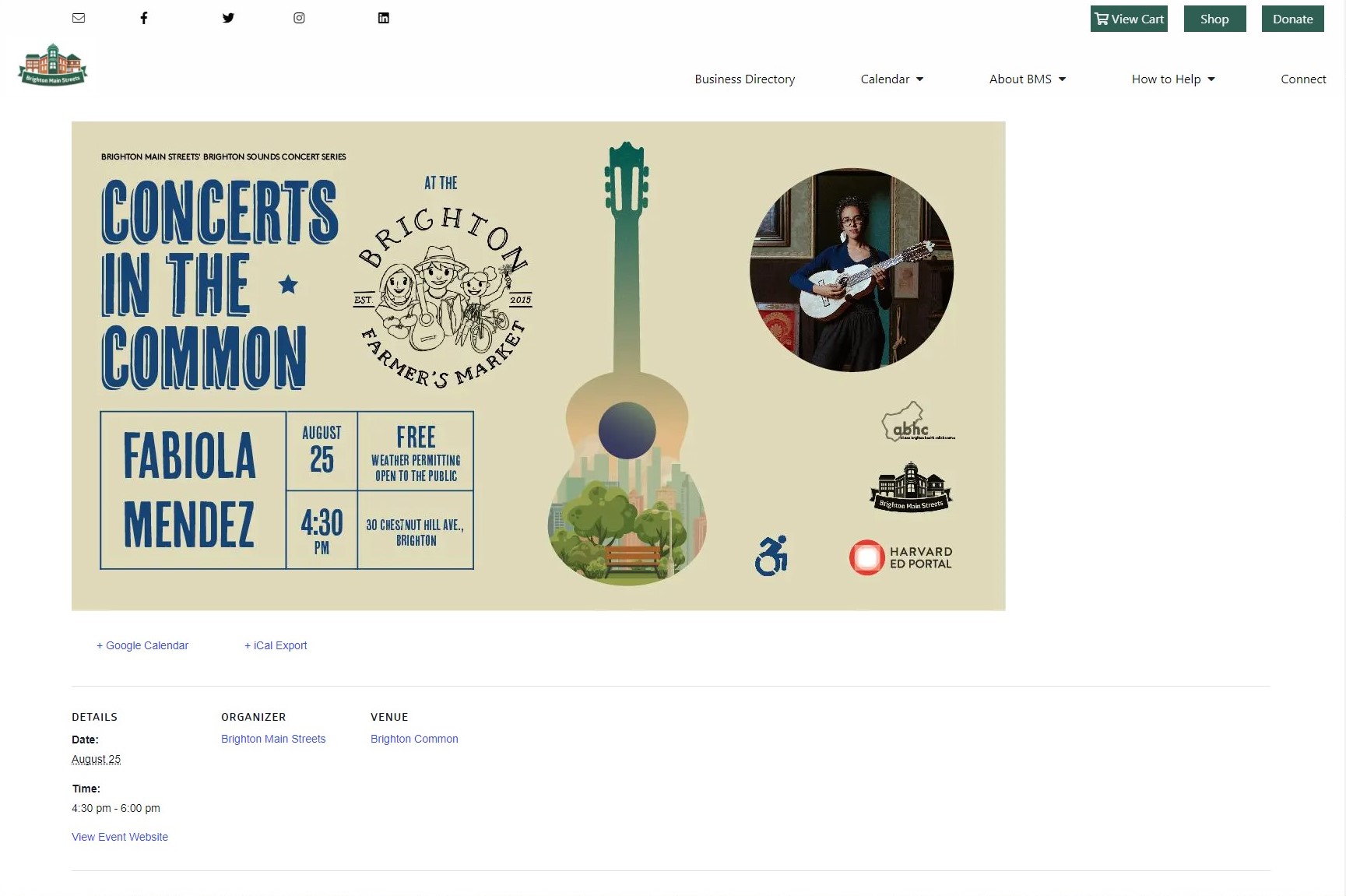This image depicts a website advertisement for an upcoming concert at the Brighton Farmers Market. The website features a clean, white background and is topped with a logo in the upper left corner resembling a schoolhouse, which is somewhat difficult to make out due to its small size. On the left side of the page, there are links to email the organization or visit their social media profiles. On the right side, options include "View Cart," "Shop," "Donate," and below these are categories like "Business Directory," "Calendar," "About BMS," "How to Help," and "Connect."

The central focus of the image is a tan-colored advertisement for the concert. The ad features blue text on the left side, providing details about the event: "Concerts in the Common," featuring artist Fabiola Mendez on August 25th at 4:30 PM, free and open to the public, weather permitting. The event will take place at the Brighton Farmers Market, and the address is listed below.

Accompanying the text, there is a cutout image of a guitar on the right side, which contains a scenic photograph of a park with a bench and trees. In the upper right corner of the advertisement, there is a photo of the artist, Fabiola Mendez, holding her guitar. Below her image, you can see the logos of the event sponsors, indicating their support. Additionally, there is an icon indicating that the event is Handicap accessible.